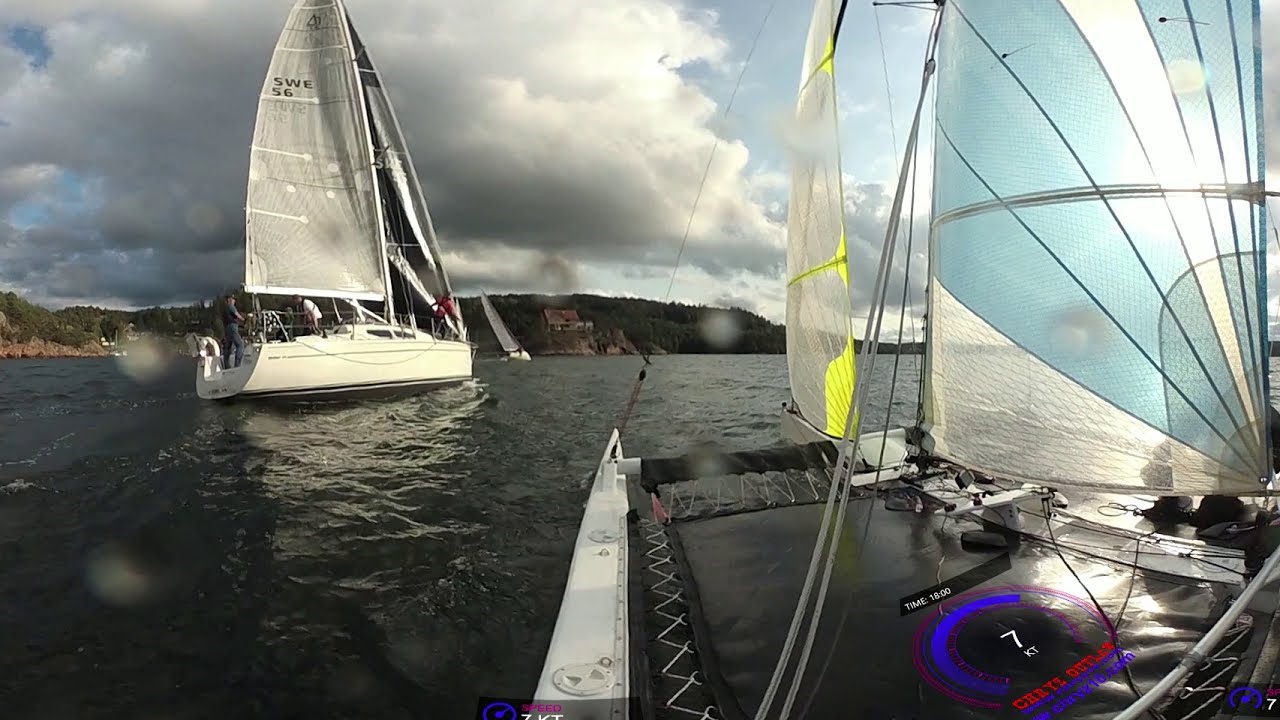In this outdoor sailing regatta scene, the focus is on two boats surrounded by a large expanse of dark, cloudy water, under a predominantly gray sky with hints of blue. In the foreground on the right-hand side, a large catamaran dominates, identifiable by its white netting and spongy trampoline deck. Its colorful sails are fully open, featuring a mix of green, blue, yellow, and white patterns, and some red and purple lettering, although partially obscured. A purple circle with white text saying "7-something" is visible among the deck details. On the left side of the image, there is another sailboat, primarily white, with its sails hoisted and catching the wind. This boat has at least three people aboard: one in blue at the stern, one mid-ship, and another in a red shirt toward the bow. Just to the right of this sailboat, in the distance, a smaller unidentified boat can be seen, leaning into the wind with its full sails open. Beyond the boats, a hilly landscape with dark green trees stretches across the middle of the picture, reinforcing the outdoor setting on this cloudy day reminiscent of a sailing competition.